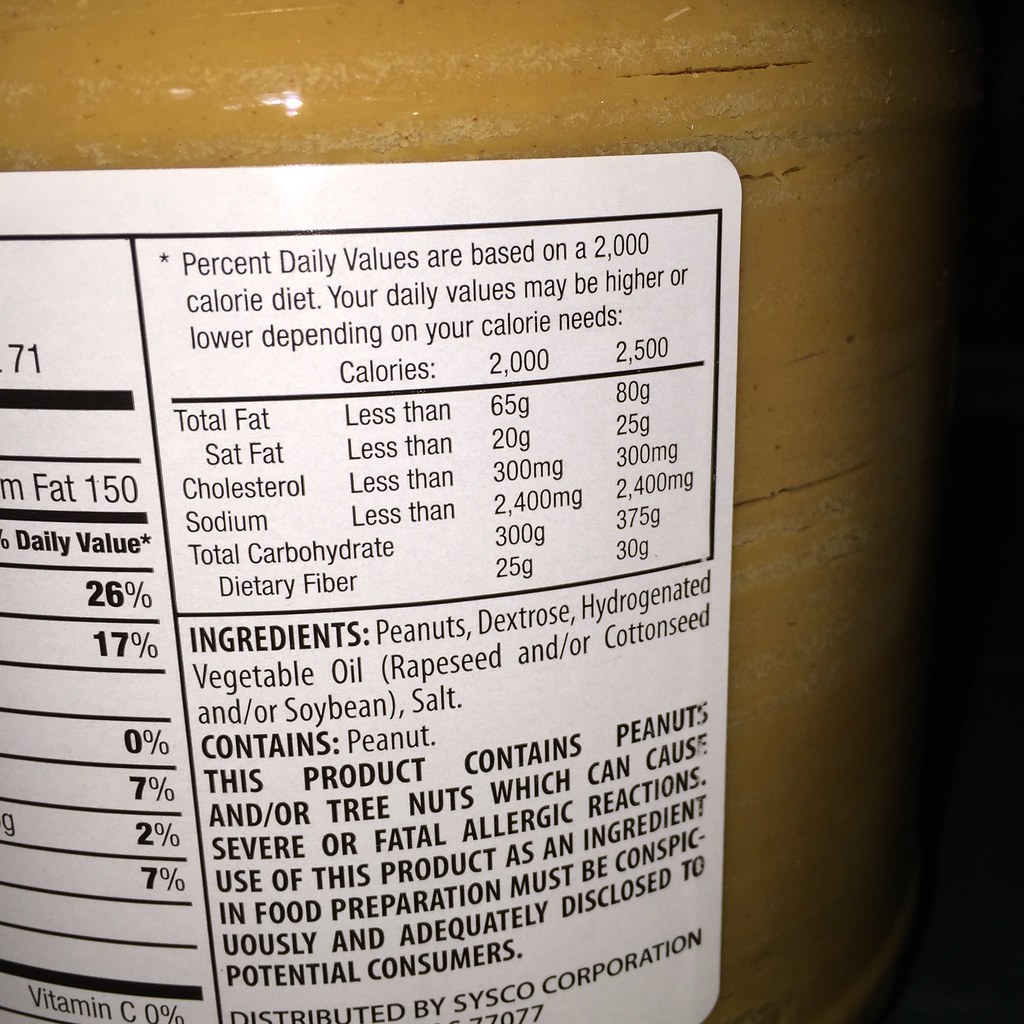The image displays a detailed ingredients label of what appears to be a jar of peanut butter. The label clearly lists "peanuts" among its prominent ingredients, indicating its primary component. The jar itself seems quite large, although the actual size might be exaggerated due to forced perspective in the photograph. The close-up photo of the label occupies just a corner of the image, providing a partial view of the overall product. The picture was taken in a dimly lit room, using flash photography, as evidenced by the bright reflection of the camera’s flash on the plastic surface of the peanut butter jar.